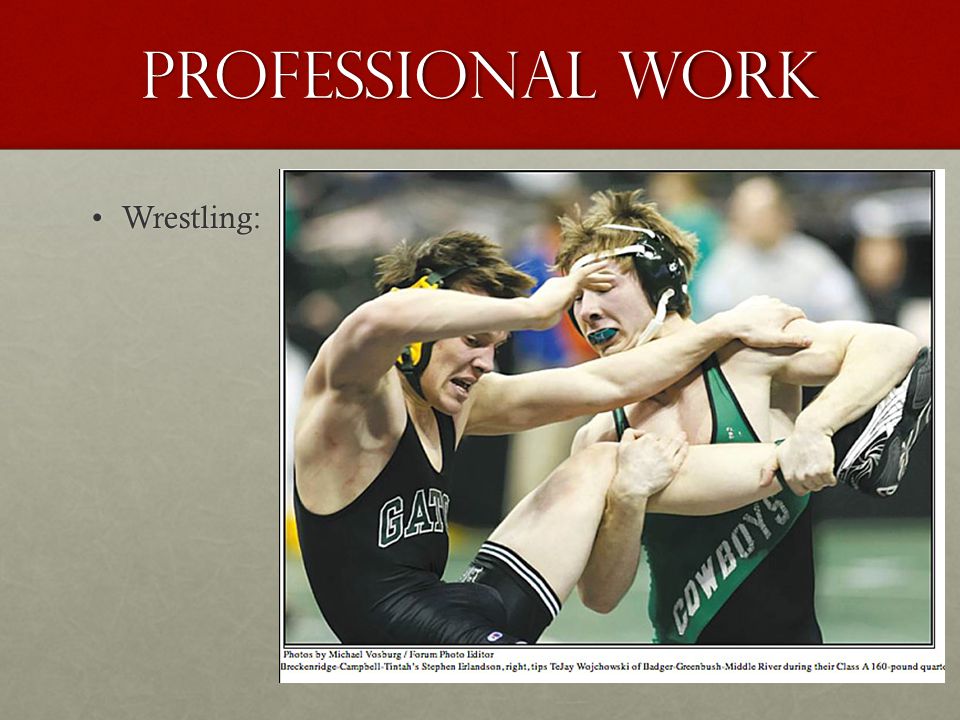The image, possibly from a newspaper article or presentation slide, prominently displays the title "Professional Work" in bold white letters across a red banner at the top. Below, the word "Wrestling" is featured, followed by a photograph capturing two male wrestlers mid-match. Both athletes are clad in singlets; one wrestler wears a half green, half black singlet with "Cowboys" inscribed on it, while the other dons a plain black singlet with the letters "GAT". Both competitors have on ear guards and mouth guards. The wrestler in the green and black singlet has his opponent’s leg hoisted in the air, seemingly about to bring him down. The photo credit, although in very small text, identifies Michael Vosburgh as the photographer. Additionally, the text below the image provides details of the athletes, categorized as Class A, 180-pound wrestlers.